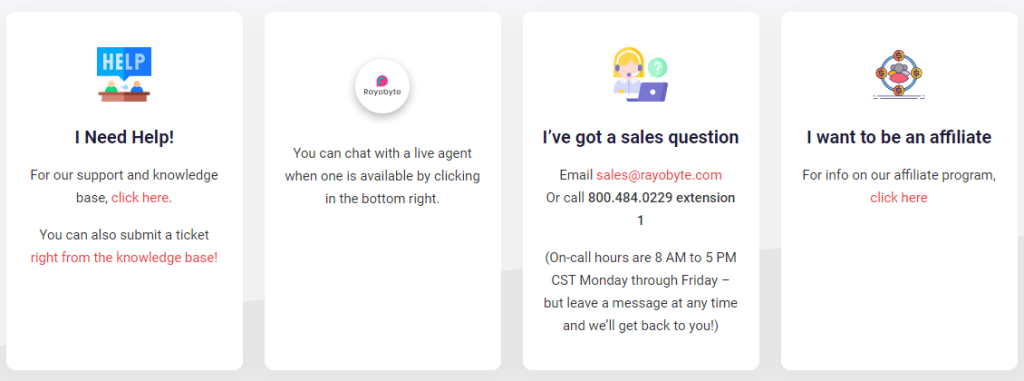This is an in-depth descriptive caption for the image provided:

"A horizontal screenshot of an online help desk interface featuring four distinct selections set against a subtle gray gradient background. Each selection is contained within vertical rectangles aligned horizontally. The first selection is labeled 'Help, I need help for our support and knowledge base.' It features a clickable 'Click Here' link that is highlighted in red text. The second section is titled 'Rayobite' and offers the option to 'chat with a live agent when one is available' by clicking the button located in the bottom right corner. The third section, labeled 'I've got a sales question,' includes a graphic of an IT person with blonde hair and headphones. Below the graphic, it provides contact information, including an email address: sales@rayobite.com, and a phone number: 800.484.0229 ext. [extension]. Additionally, it lists the on-call hours as 8 a.m. to 5 p.m. Central Standard Time, Monday through Friday, while noting that messages can be left at any time. The final section is titled 'I want to be an affiliate' and invites users to click on a red hyperlinked text for information regarding their affiliate program."